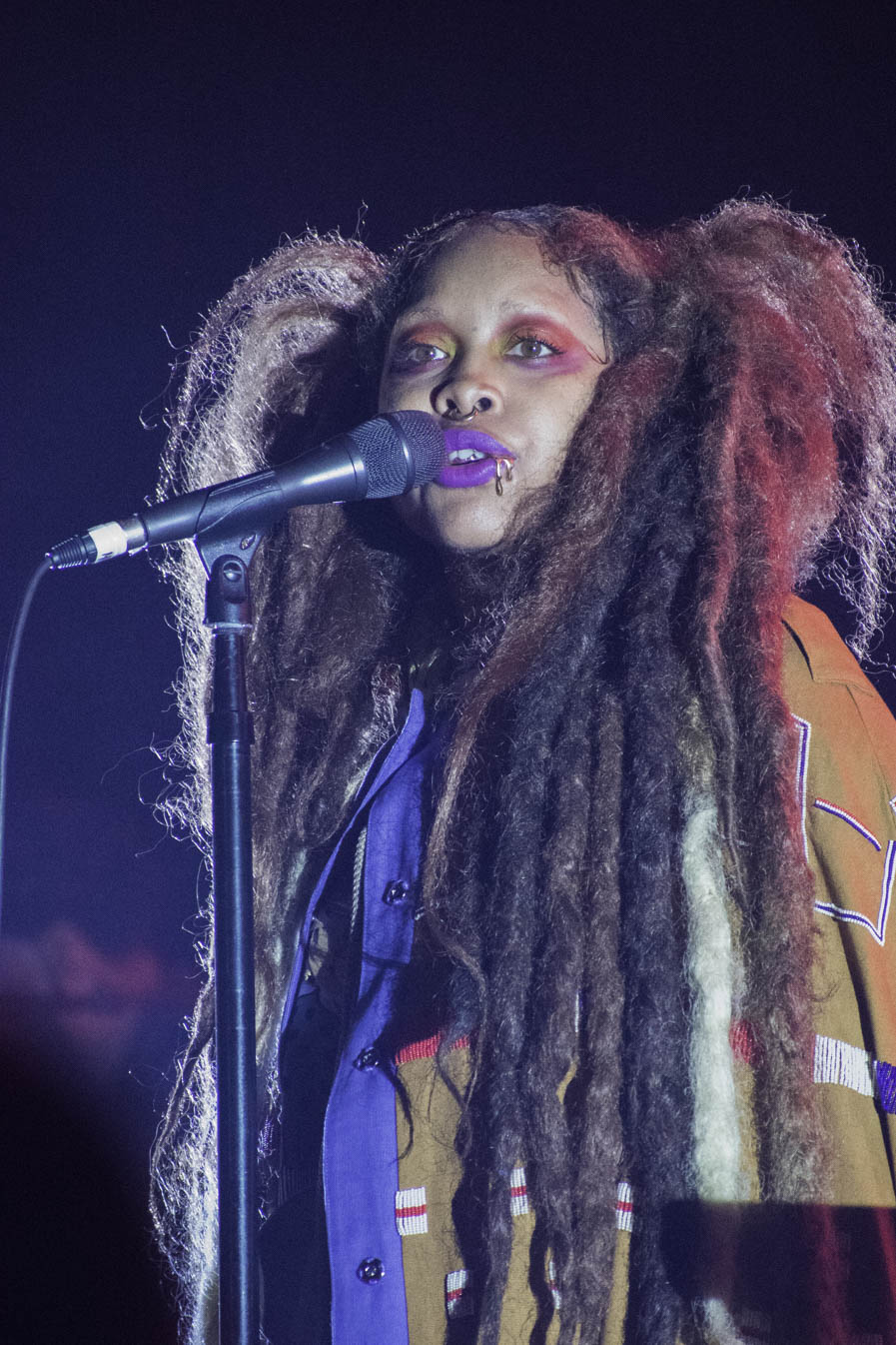This photograph captures a striking scene of a light-skinned African-American female singer, likely Erykah Badu, performing on stage. She is depicted from the torso up, with long, multicolored dreadlocks tied into pigtails that cascade down to her waist. Her face is adorned with prominent makeup including bright purple lipstick and exaggerated red and yellow eyeshadow. She has a gold nose ring under her nostrils and two gold lip rings at the bottom right corner of her mouth. She appears to be singing into a tall black microphone that is positioned to her left. Her outfit consists of multiple layers, including a light brown jacket with blue borders and beads, along with an underlying blue shirt. The stage light highlights her against a black backdrop, creating a dramatic and vivid portrait of the artist mid-performance.